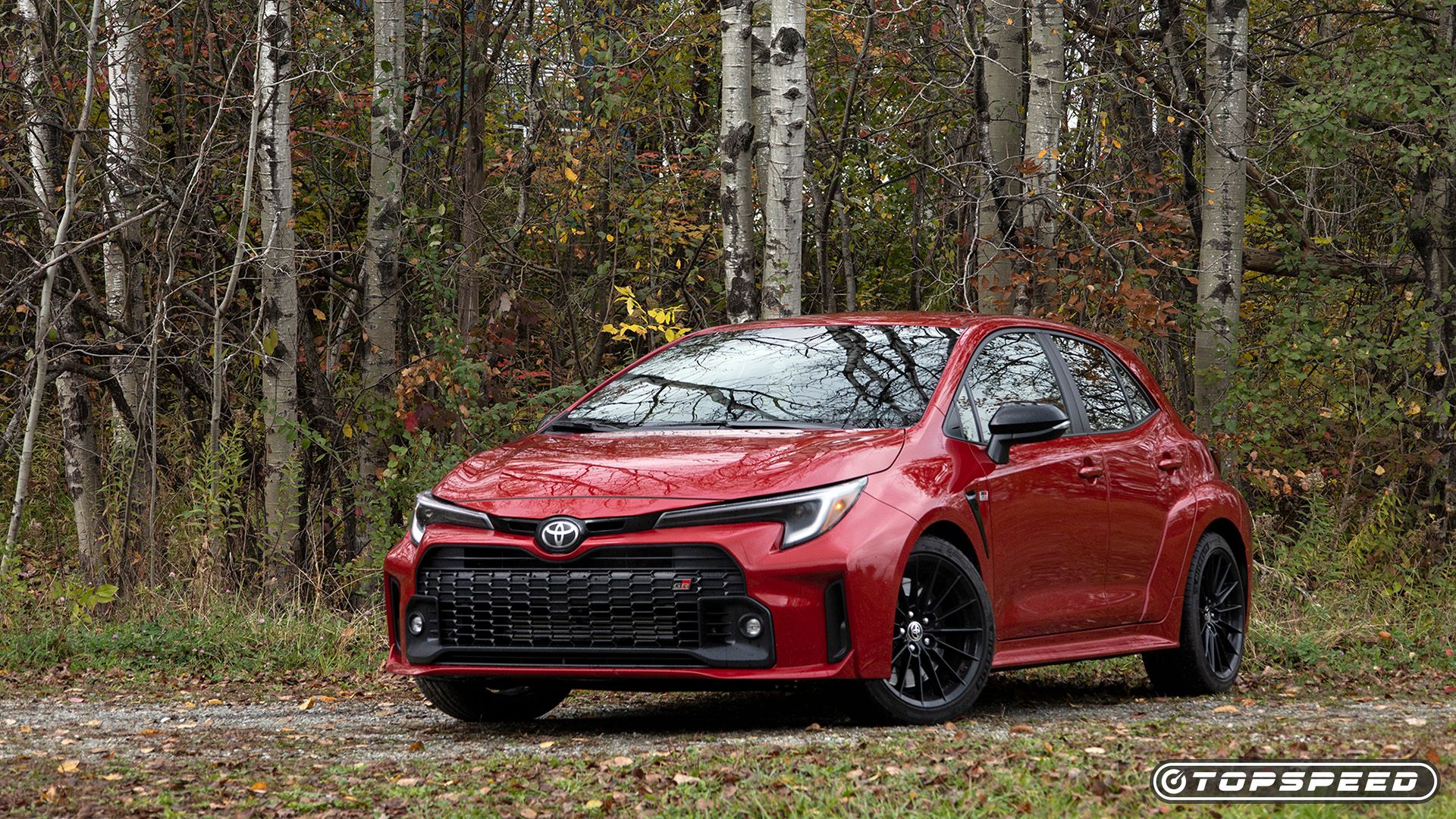This photograph features a deep red Toyota sedan with black accents, including a black grill and black rims, parked on a gravel road in a wooded area. The background is filled with trees characterized by white bark and black spots, along with a mix of green, yellow, and red leaves, and abundant fallen foliage on the ground. Reflections of the foliage and trees are visible on the car's surface. In the bottom right corner of the image, there is an oval shape with a gray background and white lettering that reads "TOP SPEED," accompanied by a small circular illustration with a line through it, possibly indicating a show or feature about cars.